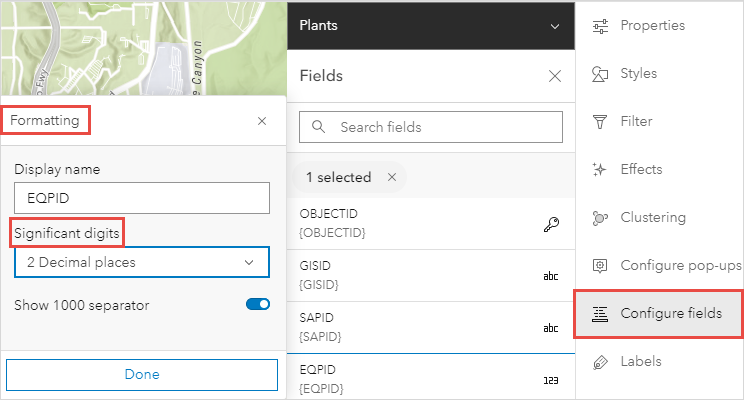**Website User Interface Description:**

The website is divided into three distinct sections:

1. **Left Section (approximately 4 inches wide):**
   - The top inch and a half displays a small segment of a map, featuring some green areas representing grass and a blue area depicting a river. The map extends approximately an inch further down towards the bottom.
   - Below this map, a white rectangle with a red border encloses the word "formatting."

2. **Middle Section (approximately 4 inches wide):**
   - Starting from the bottom and extending about halfway up is another section of water, bordered by white lines indicating roads.
   - Below this water segment:
     - There is a bold red rectangle labeled "significant digits."
     - Below this, a blue rectangle spans the entire width of the column, with the text "two decimal places" inside it.
     - Further below, the text "show 1000 separator" is followed by a blue slider with a white indicator.
     - At the bottom, a tab stretches across the width with the word "done."

3. **Right Section (approximately 2 inches wide):**
   - At the top, the section features an "X" icon.
   - Below this, the text "display name" is accompanied by a rectangle containing "EQPID."
   - Information is grouped vertically as follows:
     - "Properties"
     - "Styles"
     - "Filter"
     - "Effects"
     - "Clustering"
     - "Configure pop-ups"
     - "Configure fields" with a red border around it
     - "Labels"
   - Icons representing the aforementioned options are positioned to the left of each respective label.

**Center Section (interwoven):**
- A black-bordered rectangle with the word "plants" in white, located towards the left side.
- A white rectangle labeled "fields" also positioned towards the left.
- A search rectangle is present, with additional informational content below it.

The layout is meticulously structured with distinct borders, labels, and color-coded sections to facilitate user navigation and interaction.